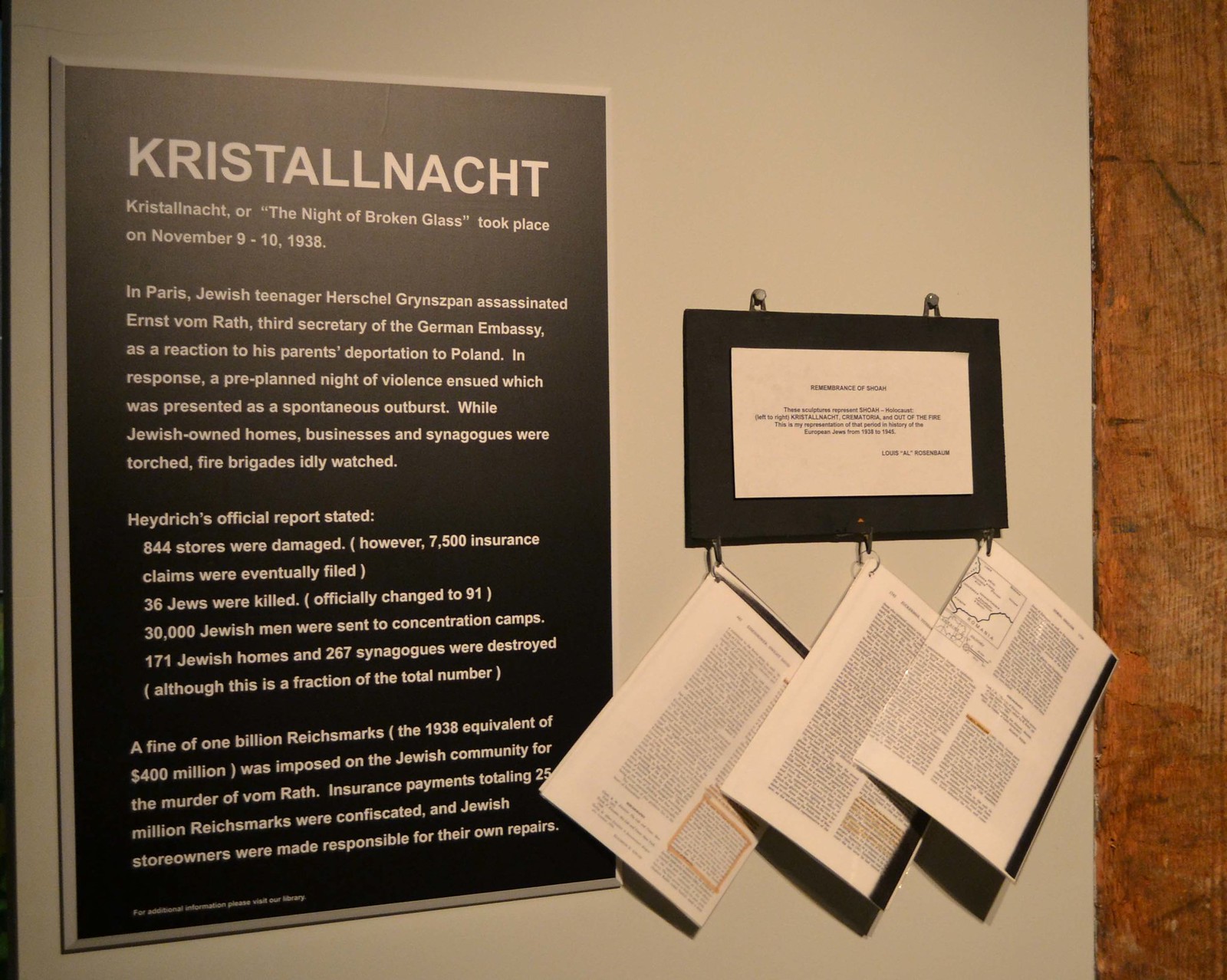The image appears to be taken inside a museum, showcasing a historical exhibit with a focus on Kristallnacht, or the "Night of Broken Glass," which occurred on November 9th to 10th, 1938. The exhibit is mounted on a light gray-colored wall, with a large black plaque prominently displayed on the left. The plaque bears the word "KRISTALLNACHT" in bold, white capital letters followed by a detailed explanation of the event in multiple paragraphs of white text. To the right of this main plaque, there is a smaller framed rectangle outlined in black, holding a piece of white paper that includes black text, though it's too small to read clearly. Attached to the bottom of this smaller plaque are three folded pages or booklets, also featuring dense black lettering with some highlights in orange, though the specifics are not legible. The wall extends from left to right across the image, with a small section of a brown wooden surface visible on the far right side. The hanging booklets are aligned slightly askew, with their tops angled towards the right and their bottoms towards the left, partially overlapping each other. This setup provides additional information and context for the main exhibit plaque.